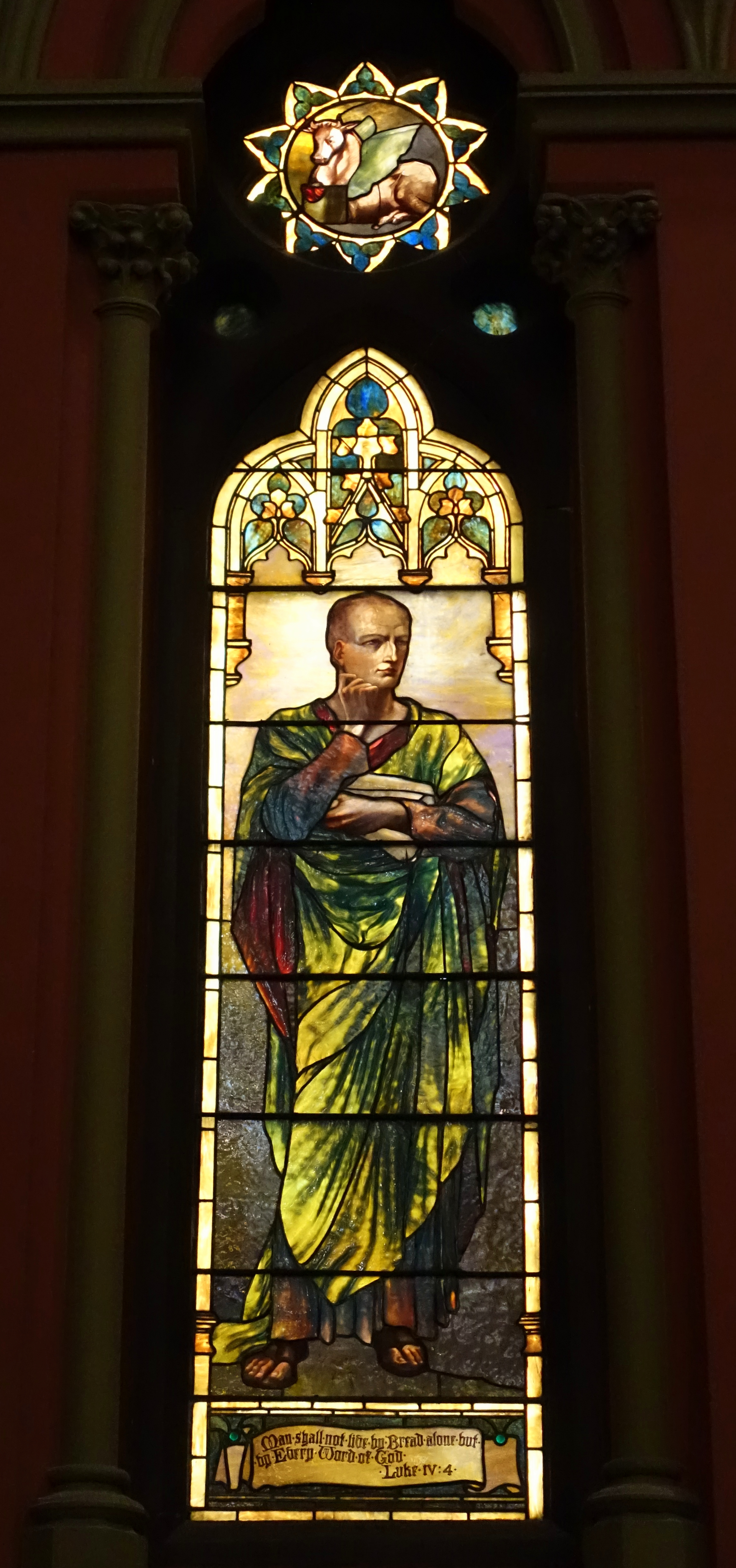The image portrays an ornate stained glass window, set in a red wall adorned with brown crown molding. Framing the window are vertical pillars, enhancing its architectural elegance. At the very top of the structure is a circular stained glass design featuring a sun, outlined in green and blue patterns, with a unique depiction of a cow with green wings in the center.

The main focus of the window is a robed man, possibly a religious figure. He appears to be balding and is gazing forward and slightly to his right. He stands in a yellowish-green robe with dark sleeves and brown sandals. Under his left arm, he seems to hold papers or a scroll, and his hand is placed thoughtfully under his chin. Behind his head, intricate and colorful designs add further detail to the scene.

At the bottom of the window, within a small rectangle, there is an inscription that reads "Man shall not live by bread alone but by every word of God," followed by "Luke 4:4." Above the figure's head, more stained glass designs in green, blue, and yellow further embellish the window. The entire window culminates in a rounded arch at the top, giving it a distinguished and elaborate appearance.